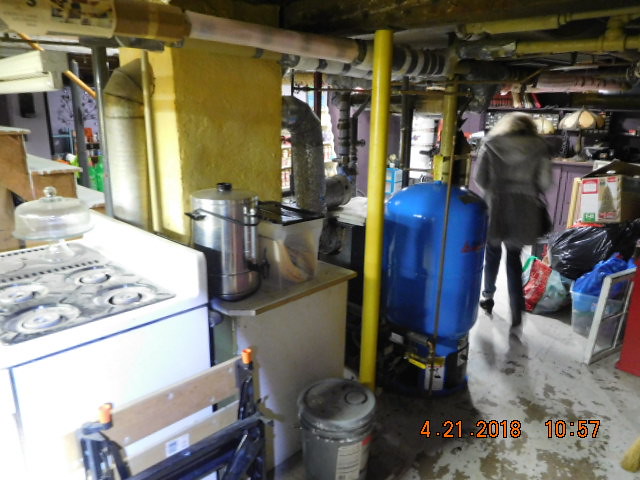The image, dated April 24th, 2018 at 10:57 a.m., depicts a cluttered basement or underground storage area, potentially linked to a restaurant due to the presence of various kitchen items and industrial equipment. The floor is concrete with chipping paint, and numerous large blue and yellow pipes run along the ceiling and walls, hinting at an industrial setting. Prominent features include a large blue gas cylinder and a noticeable yellow column with attached pipes. Among the scattered items, there's an old white stove with a glass cake container atop it, numerous large aluminum cooking pots, possibly for more than just culinary use, and a portable Black & Decker workbench. The space is filled with miscellaneous storage boxes, old mechanical equipment, mess, and garbage. In the scene, a woman in a grey coat is seen from behind, walking away towards a brighter exit, past various discarded plastic bags.